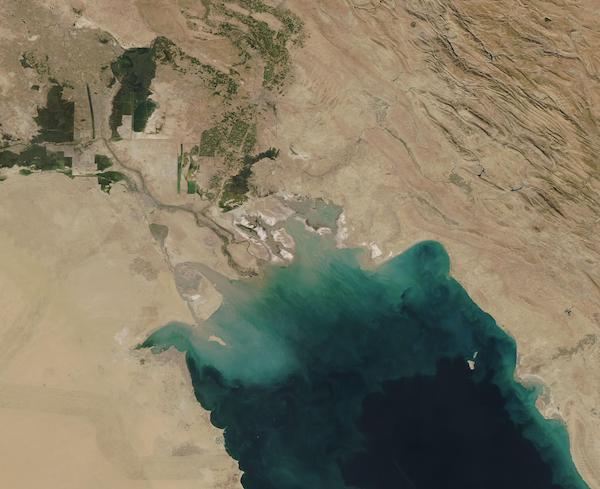This aerial photo captures a strikingly arid landscape dominated by an almost desert-like lake. The lake, an ombre mix of dark teal that fades into tan as it stretches, starts in the bottom right of the image and angles towards the upper left, extending only a few inches into the frame. The lake's deep emerald green waters create a stark contrast against the surrounding barren brown dirt. To the right and left of the lake, the land remains lifeless and parched. However, just above the lake, patches of green vegetation cling to the arid earth, appearing more concentrated and vivid as they spread outwards. Different textures on the right side of the photo suggest varied elevations or possibly mountainous terrain, contributing to the desolate beauty of this dried-up landscape that might even resemble the Euphrates region.